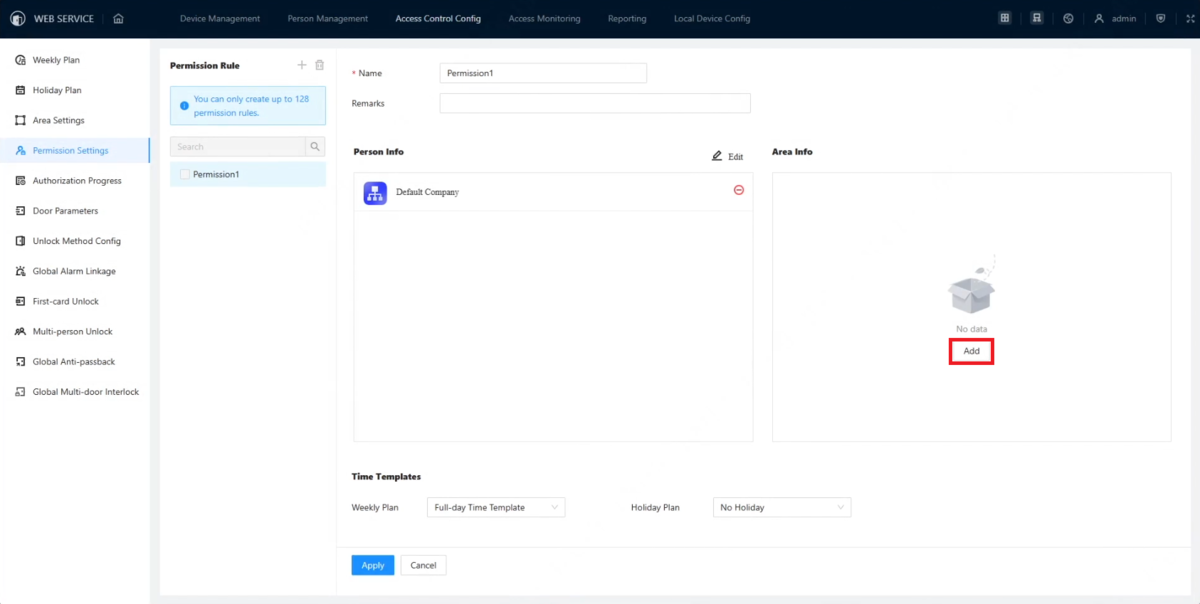Screenshot of a web service interface: 

At the upper left-hand corner of the screen, the words "WEB SERVICE" are displayed in capital white letters accompanied by a logo positioned to their left. These elements are embedded within a thin black ribbon that stretches horizontally across the top of the page. Proceeding to the right, there are several navigation options, including a home icon followed by menu items such as "Device Management" and "Person Management," though some of the text is too small to discern clearly.

The central portion of the screen features a white background. A vertical list of options is situated on the far left side, each item rendered in gray text and paired with appropriate icons. This list includes selections such as:
- Weekly Plan
- Holiday Plan
- Area Settings
- Permission Settings
- Authorization Progress
- Door Parameters
- Unlock Method Config
- Global Alarm Linkage
- First Card Unlock
- Multi-Person Unlock
- Global Anti-Passback
- Global Multi-Door Interlock

To the right of this vertical menu, the top part of the main display showcases the bold black text "Permission Rule." Below this heading is a light blue box containing the information "You can only create up to 128 permission rules" in bright blue text. Underneath this notification, there is a short, gray search bar.

Further down, the interface presents another light gray box labeled "Permission One" in gray text. To the right of this label, multiple interactive boxes provide additional functions integral to managing permissions within the web service system.